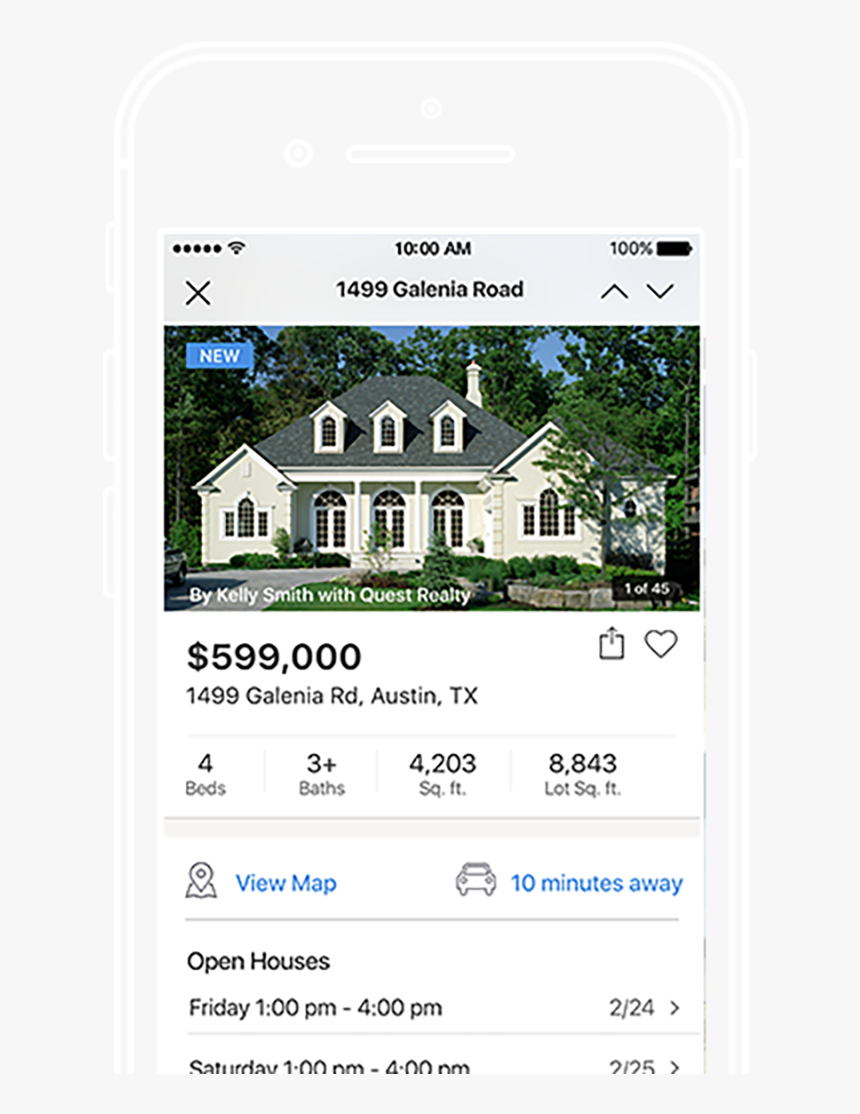This image is a detailed screenshot from a real estate app, potentially Zillow or a similar platform, framed within a white wireframe placeholder designed to resemble an iPhone. The outer border of this frame is gray, while the screenshot itself is in full color. 

At the top of the app's interface, the header displays the address "$14.99 Galenia Road." Directly below the header is a high-resolution image of a single-story, white stucco home with a gray tiled roof, evocative of classic single-family homes. 

Further down, the listing information is presented in a white font: "Buy Kelly Smith with Quest Realty." Beneath that, the price of the house is prominently listed at "$599,000." The address is reiterated as "1499 Galenia Road, Austin, Texas."

Accompanying this primary information, additional details reveal that the house comprises four bedrooms, three baths, and spans an area of 4,203 square feet. Information about upcoming open houses is also available, with one scheduled for February 24th from 1 PM to 4 PM.

The app interface suggests that users can swipe through the images to view more photos of the house and possibly access further information about the property.